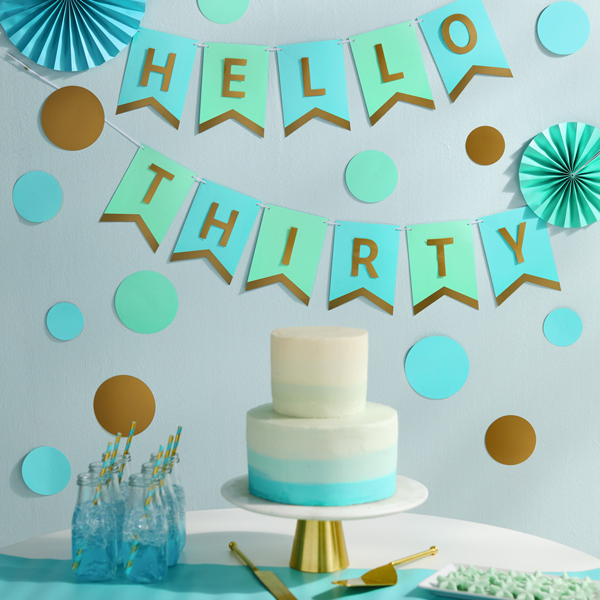This detailed image is a 3D color illustration, likely created using a program such as SketchUp, depicting a sophisticated birthday celebration setup. Central to the scene is a two-tiered birthday cake presented on a white marble platter with a brass conical base. The cake, intricately designed, features a smaller white top tier and a larger base tier adorned with gradient bands transitioning from white to light blue and then darker blue. The elegant display occupies a white round table partially draped with a light blue tablecloth, contrasting beautifully with the gold metal cylindrical support of the cake stand.

To the left of the cake, there are six clear bottles filled with water, each fitted with a golden and light blue straw, contributing to the cohesive color scheme. Directly in front of the cake, a gold cutting knife and spatula rest, ready for slicing. On the right side, a small rectangular plate holds an assortment of cookies.

The backdrop enhances the festive atmosphere with a pennant banner spelling out "Hello 30" in brown letters on blue and green flags. The wall showcases a mixture of dark brown and aqua circles interspersed with decorative fan circles, adding depth and vibrancy to the scene. This visually appealing composition highlights the cake as the focal point, accentuated by thoughtfully arranged decorations and serving items.